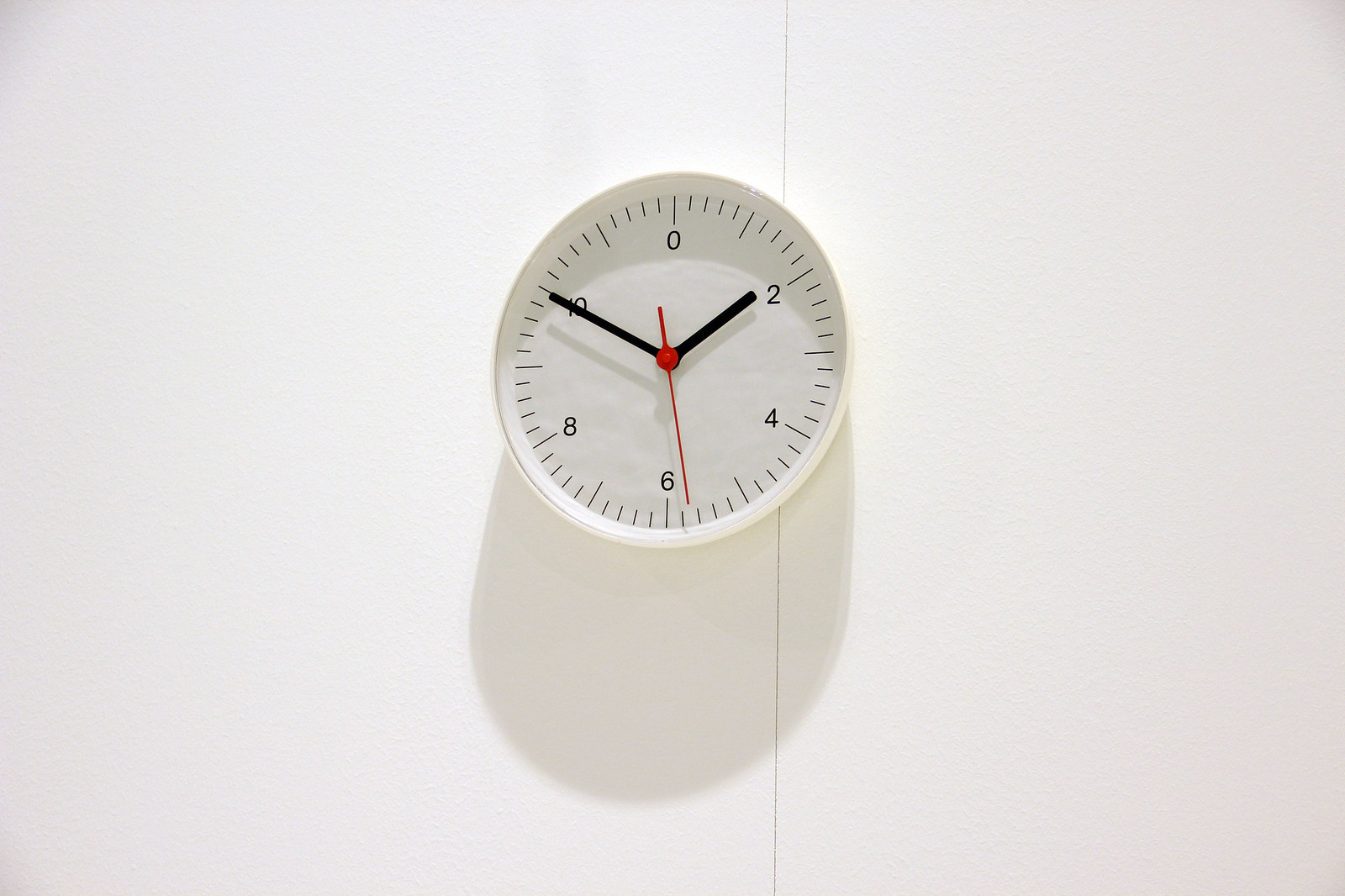In this indoor color photograph, a simplistic, round, plastic wall clock is mounted on an off-white wall. The wall features a thin vertical line running from top to bottom, slightly to the right of the clock, which is positioned just to the left of the line. The clock itself has a white background with a white rim. It features black hour and minute hands, and a red second hand. The time displayed is 2:50, with the minute hand just before the 6 o'clock position and the hour hand on the 2. Instead of a traditional 12 at the top, the clock has a 0 at the 12 o'clock position, with other numbers reading 2, 4, 6, 8, and 10, separated by small slashes on the outer rim. Additionally, there is a shadow cast by the clock, indicating a bright light source from above.